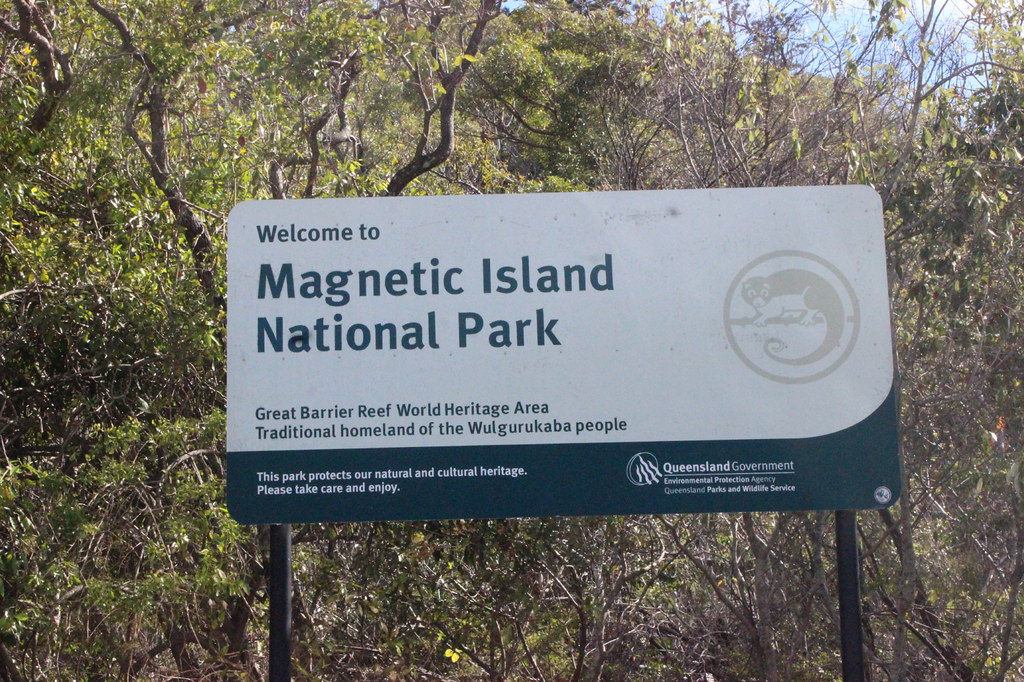This horizontal image features a prominent sign welcoming visitors to Magnetic Island National Park, a part of the Great Barrier Reef World Heritage Area and the traditional homeland of the Ulgarubabkaba people. The sign is predominantly off-white, with a lower green section that swoops up on the right side. On the off-white portion, green lettering provides information about the park. The lower green section, with white lettering, emphasizes the park's role in protecting natural and cultural heritage, urging visitors to take care and enjoy their experience. 

On the right side of the sign, there is an emblem featuring a long, curled tail symbol. The green section also includes the logos and names of the Queensland Government Environmental Protection Agency and Queensland Parks and Wildlife Service. The sign stands mounted on two sturdy 4x4 posts. 

In the background, the dense thicket of thick trees and brush is visible, with a small patch of blue sky peeking through the upper right corner, highlighting the lush and vibrant forest that surrounds this rectangular sign.